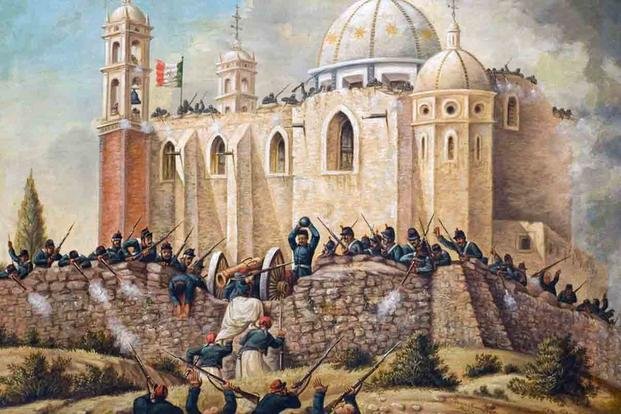The colored drawing showcases an intense battle scene set during what appears to be a medieval era, featuring a large, rectangular castle with defensive structures and soldiers actively engaging in combat. The castle, likely influenced by Islamic architectural elements, is characterized by its multiple arched windows, corner towers, and a prominent white dome adorned with yellow stars at its center. A cross and stars crown the building, suggesting a fusion of religious symbols.

At the forefront of the scene, soldiers clad in blue tunics, blue caps, and white bandoliers defend a short, slightly curved stone wall. One notable detail is a bronze and white cannon strategically placed in a dip of the wall, aimed downward towards the attackers. Among the defenders, one man is wielding a cannonball above his head, ready to hurl it down at the opposing force. Another man, already struck, leans over the wall.

The attackers, seen climbing up the hill towards the castle, are dressed in loose white pants, blue jackets, and red caps. The scene includes details such as a tree on the left side and a background filled with gray, cloudy skies, likely from the smog and blasts of the ongoing battle. A flag, which could be green, white, and orange, belonging possibly to Mexico or Ireland, adds an element of nationality to the conflict. The entire composition underscores the chaos and ferocity of the siege, with both sides fiercely engaged.